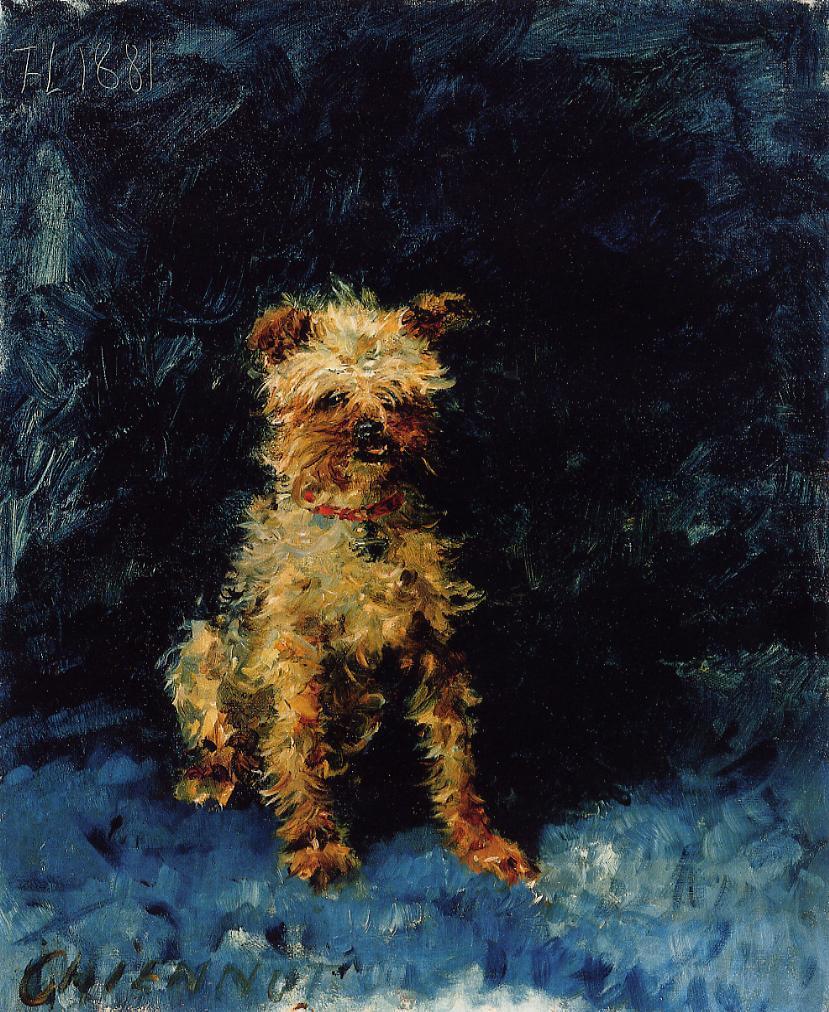This oil painting portrays a cute, small to medium-sized scruffy dog in a sitting position, created with wild, impressionistic, yet realistic brushstrokes. The dog features a mix of light brown and dark brown fur, with a few beige highlights and shades of black, particularly around his eyes, nose, and face. His fur displays various tufts and scruffy patches, with a hint of orange on his paws. He sports a red collar adorned with a slightly visible silver emblem or large silver bell. His black eyes and nose stand out prominently, and his mouth is slightly open. The background transitions from a powder blue carpet at the bottom to a deep midnight blue at the top, painted with thick, textured strokes. On the bottom left-hand side, the inscription "Chino" (C-H-I-E-N-O-T) is visible, while the top left-hand corner features the marking "FL 1881" in white.